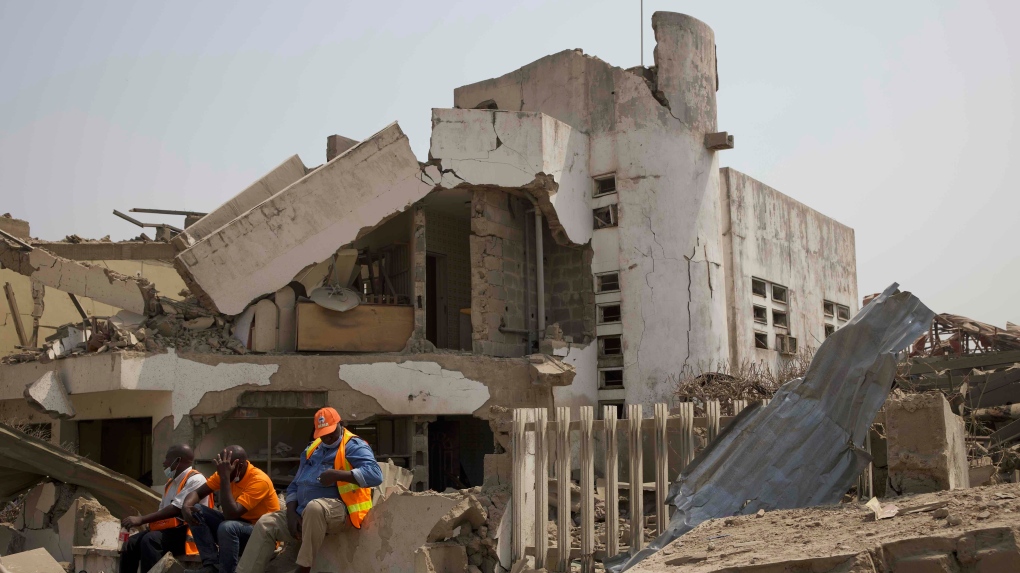The image depicts a rectangular photo of a heavily damaged concrete building, likely the result of a bombing or an earthquake, as it lies in shambles with its left side crumbling and a loose tin metal roof hanging precariously. The background is characterized by a dark, overcast sky, possibly filled with smoke or indicative of a cloudy day. In the foreground, there are three African-American construction workers, donned in bright orange safety gear, taking a break amid the rubble. The first worker, seated on the rocks, wears an orange cap, blue shirt, khaki pants, and an orange vest. The second worker, dressed in an orange shirt and jeans or pants, has his hands on his head, potentially looking frustrated. The third worker is in an orange vest and shirt with pants, similarly seated on the debris. This scene suggests an active demolition site or the aftermath of a natural disaster, with visible construction equipment in the background adding to the chaotic landscape.